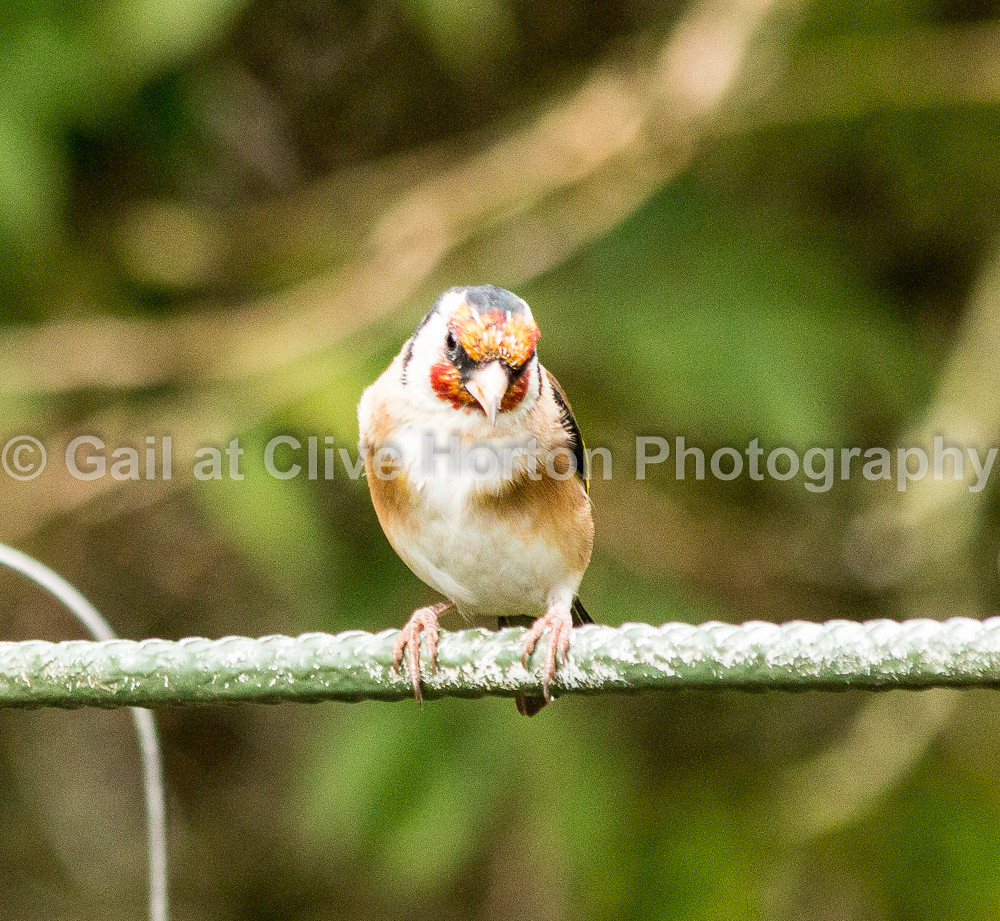This photograph captures a vivid and detailed portrait of a small bird perched on what appears to be a white rope extending horizontally across the image. The bird, centrally positioned, faces forward with its head cocked slightly to the right. Its striking plumage includes a blend of blue and red feathers on its head, complemented by a yellow beak and red feathers beneath. Its body features a mix of white and brown, while its claws, each sporting three toes, grasp the rope firmly.

Despite the bird's detailed depiction, the background is a blurred mosaic of green, suggesting trees and branches. The image is watermarked with "Gale at Clive Horton Photography" in faint white lettering, which is emblazoned near the bird's upper body along with a small symbol, possibly a copyright mark. The combination of the bird's vibrant colors and the blurred, natural backdrop creates a striking contrast, capturing the viewer's attention. The bird's complex coloration, including black around the eyes and a pale beak, adds to its unique appearance, suggesting it is a rare species rather than a common robin, blue jay, or cardinal.